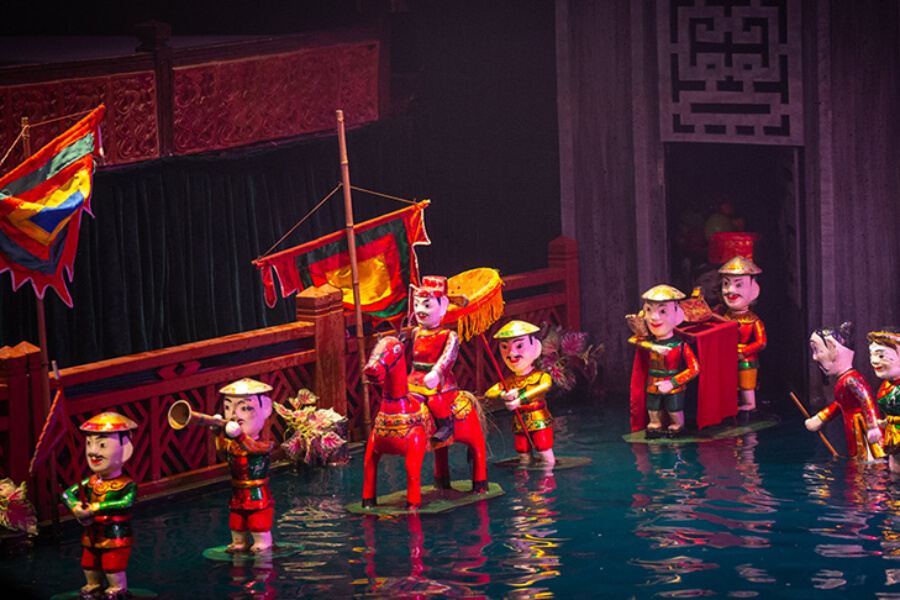In this detailed image, we see an elaborate setup featuring small figurines that appear to be floating on water. The scene includes several characters adorned in vibrant green, red, and yellow uniforms, some wearing hats. At the forefront, a figurine dressed in green with red pants and a rice paddy hat is distinguished by a mustache. Behind him, another figure in a similar outfit is playing a trumpet. Following them is a red horse with ornate decorations, ridden by a man dressed similarly to the first two. Another figurine behind the horse appears to be holding an umbrella or fan, providing shade or care for the rider. In the background, multiple colorful flags in blue, yellow, red, and green create a festive atmosphere. To the right, there are two figures carrying a square box or gift, with a woman and a child observing the scene from the far right. A red railing and an entranceway are also visible, adding to the intricate details of the tableau. The setup, filled with animated poses and diverse characters, is likely meant to depict a celebratory or ceremonial procession.